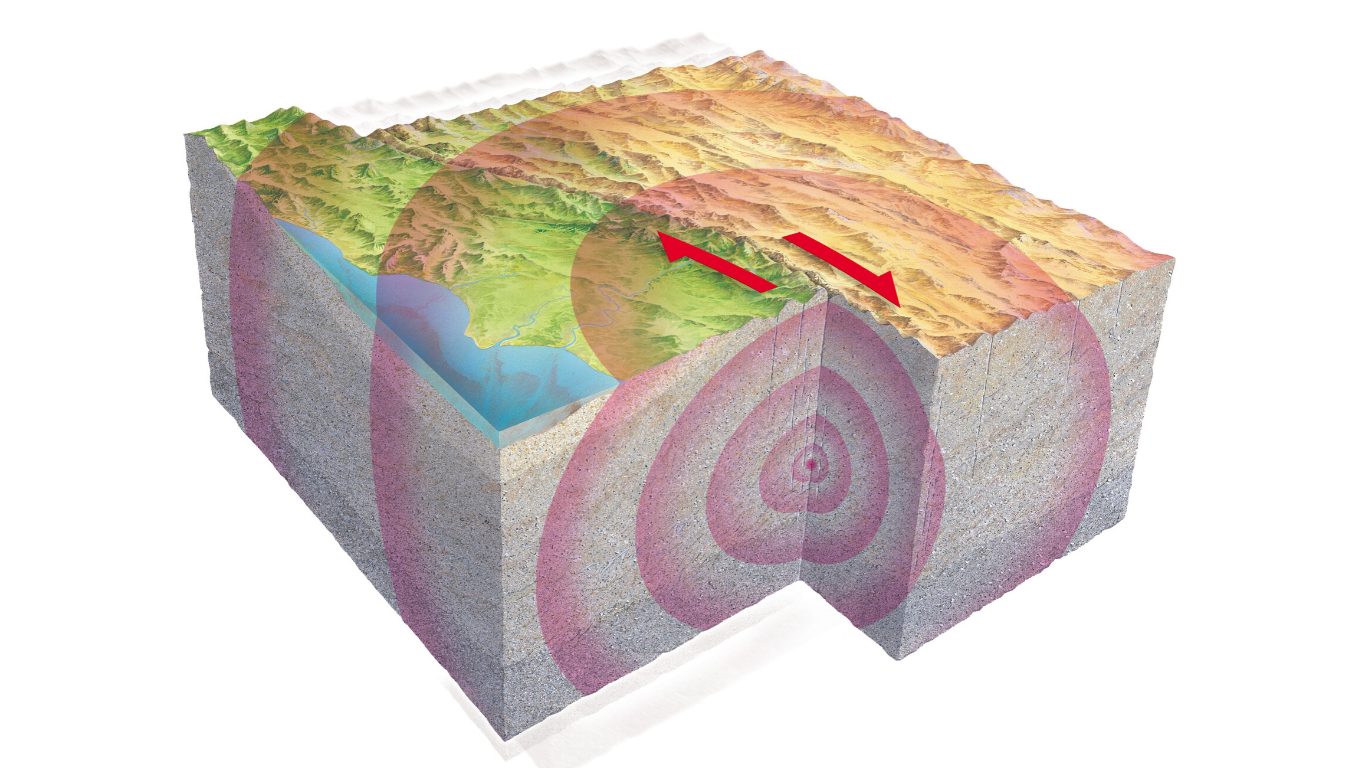This color illustration is a detailed landscape-oriented diagram depicting an earthquake's effect on the earth's crust. The diagram shows a 3D cross-section of the terrain, divided into two distinct sections along a fault line, with red arrows indicating the opposing movements of the tectonic plates. The left section is elevating, while the right section is descending, both evidenced by the arrows and visual displacement. The surface of the terrain is a topographical map where the left side is predominantly green with a water body in the bottom left corner, transitioning to the right which is mostly yellow.

The illustration reveals the layered subterranean soil, colored light gray with black specks. A series of concentric circles emanates from a central pink circle, marking the earthquake's epicenter, representing the spread of seismic waves throughout the entire section. These concentric circles highlight the areas affected by the quake. The diagram is set against a white background, clearly illustrating the geological shifts and the dynamics of tectonic plate movements in a visually engaging and informative manner.